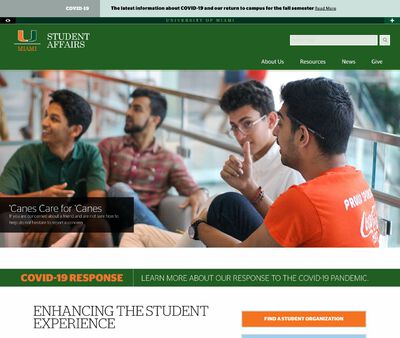The opening page of the University of Miami's Student Affairs section features a prominent orange and green "U" logo with "Miami" written beneath it. The page title reads "Student Affairs," and there is a search bar positioned on the right side of the page. At the bottom of the page, the phrase "Enhancing the Student Experience" is displayed, with an orange link to find a student organization. 

In the center of the page, there is a large photograph depicting four gentlemen engaged in conversation while seated. They have medium to dark complexions and are all sporting dark hair. Two of the men are gazing over their right shoulders. One is wearing a green shirt, another a plaid shirt, the next a white shirt, and the last is in an orange shirt. The image is accompanied by text that includes variations of the word "Care," emphasizing a supportive and attentive atmosphere.